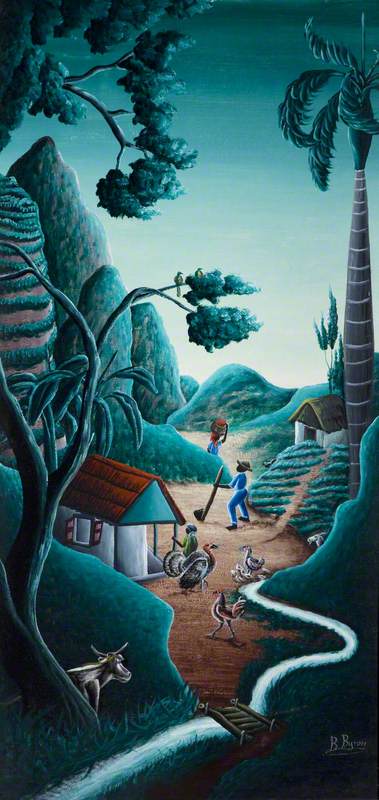The image is an illustration, possibly computer-generated or painted, with an approximately 1:2 vertical ratio. The dominant palette features greenish-blue tones, giving the scene a dark, moonlit ambiance. The setting appears to be a rural village, framed by tall trees, mountains, and cliffs. 

In the foreground, a dirt road runs through the center, leading into the hills. It crosses over a wooden bridge, and there's a mountain goat in the lower-left corner. On the right side, a towering palm tree dominates the upper part of the image. Scattered throughout the scene are several small huts, one with a red roof and white body, and another with a red and green roof. Alongside, there are various trees, including some palm trees, and small bushes and plants.

Inhabitants of the village are depicted going about their daily activities. There are several people visible: one on a bicycle in the foreground, another holding an instrument like a hoe further back, and additional figures appearing as small dabs of paint. The scene also includes animals such as a cow behind a tree in the foreground, two chickens or birds, and possibly some turkeys. The overall image exudes a feeling of a secluded, serene village enveloped in soft, muted green shades under a tranquil sky.